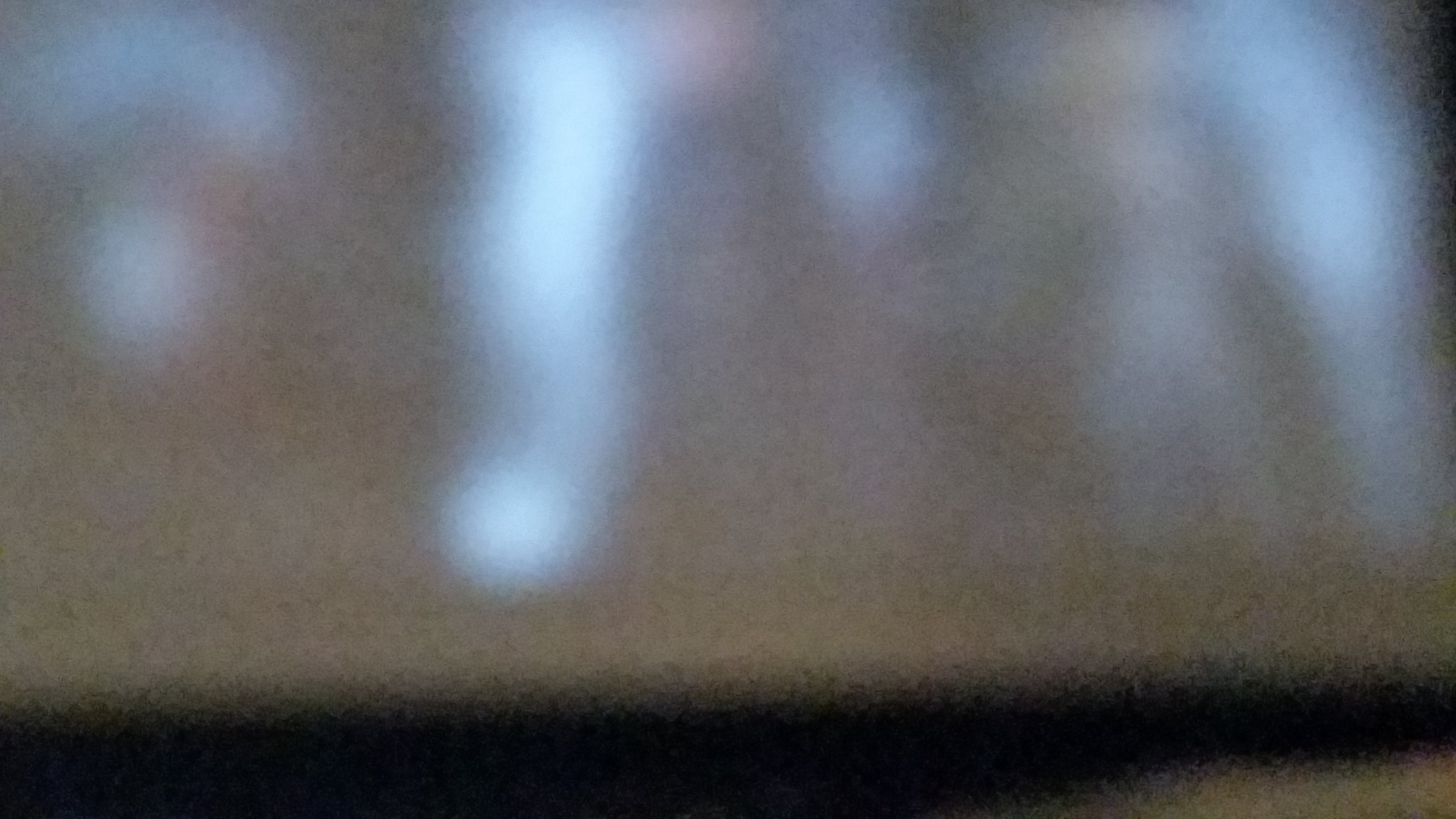This photograph depicts a fuzzy and grainy image of a television screen. The picture is awash with a bluish-white glow, making it difficult to discern specific details. However, the vague outlines of two human figures are visible, with faint skin tones indicating the positions of their heads. There is a subtle play of gray, blue, and faint red shadows on one side of the screen, adding to the overall obscurity. In the foreground, a ledge of indefinite gray-brown color is discernible, though no further details can be extracted from it. The image lacks any visible text or other distinguishable elements.